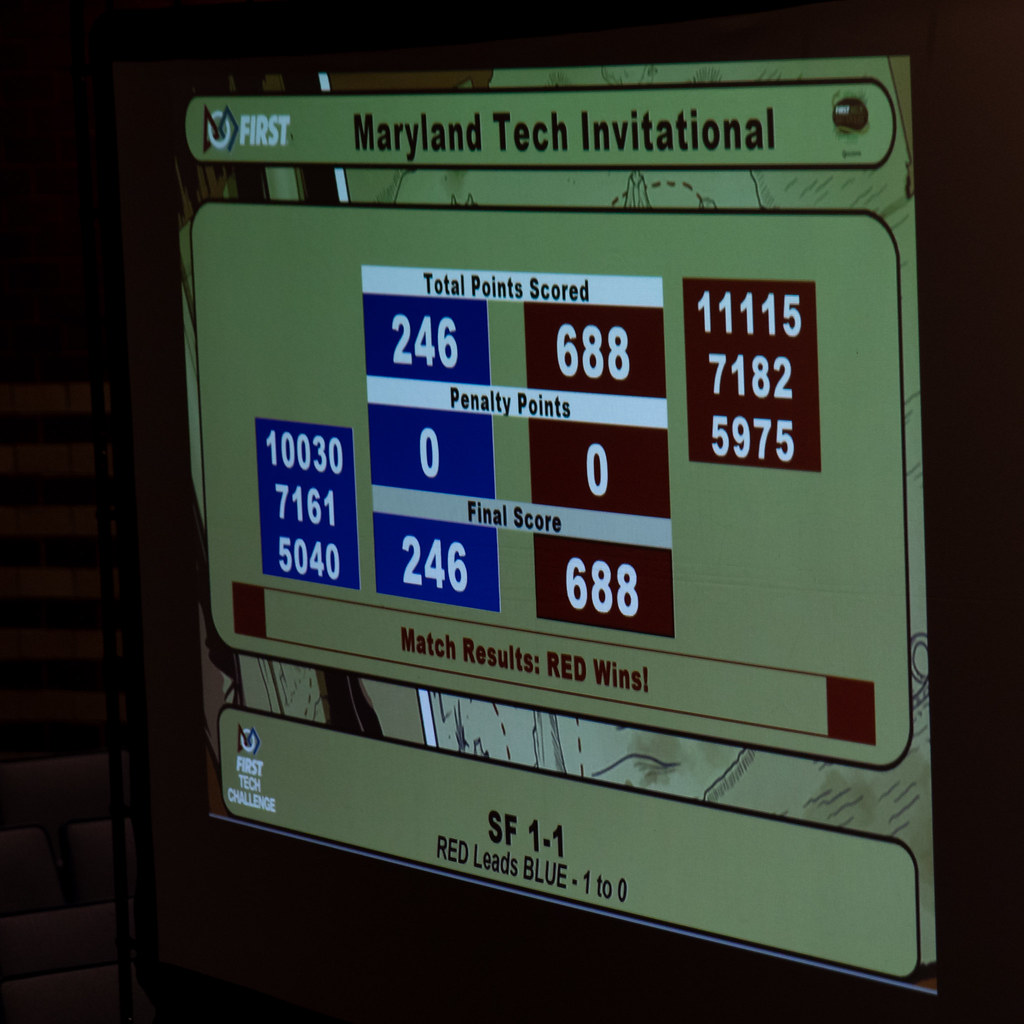The image depicts a night-time photo of a scoreboard set against a dark background. The scoreboard, primarily green with various colored highlights, prominently displays the heading "Maryland Tech Invitational" at the top. In the top left corner is the FIRST logo followed by a white rectangle that reads "Total Points Scored." Below this heading, the scores are divided into blue and red (appearing brownish in the dim light), with "246" points in a blue box and "688" points in a red box. Next, it lists "Penalty Points" as "0" in both blue and red boxes. At the bottom of this section, "Final Score" reiterates the same points: "246" in the blue box and "688" in the red box. 

On the left side of the scoreboard, there is a vertical column of blue boxes displaying the numbers "10030," "7161," and "5040." On the right side, a vertical column of red boxes shows "11115," "7182," and "5975." Below this, a strip reads "Match Results: Red Wins," indicating the red team (though the box appears brown due to lighting) has won. Finally, the bottom-most box features a rounded rectangle with the text "SF-1: Red Leads Blue, 1-0," accompanied by a logo of red and blue colors with a white circle center, reading "FIRST Tech Challenge."